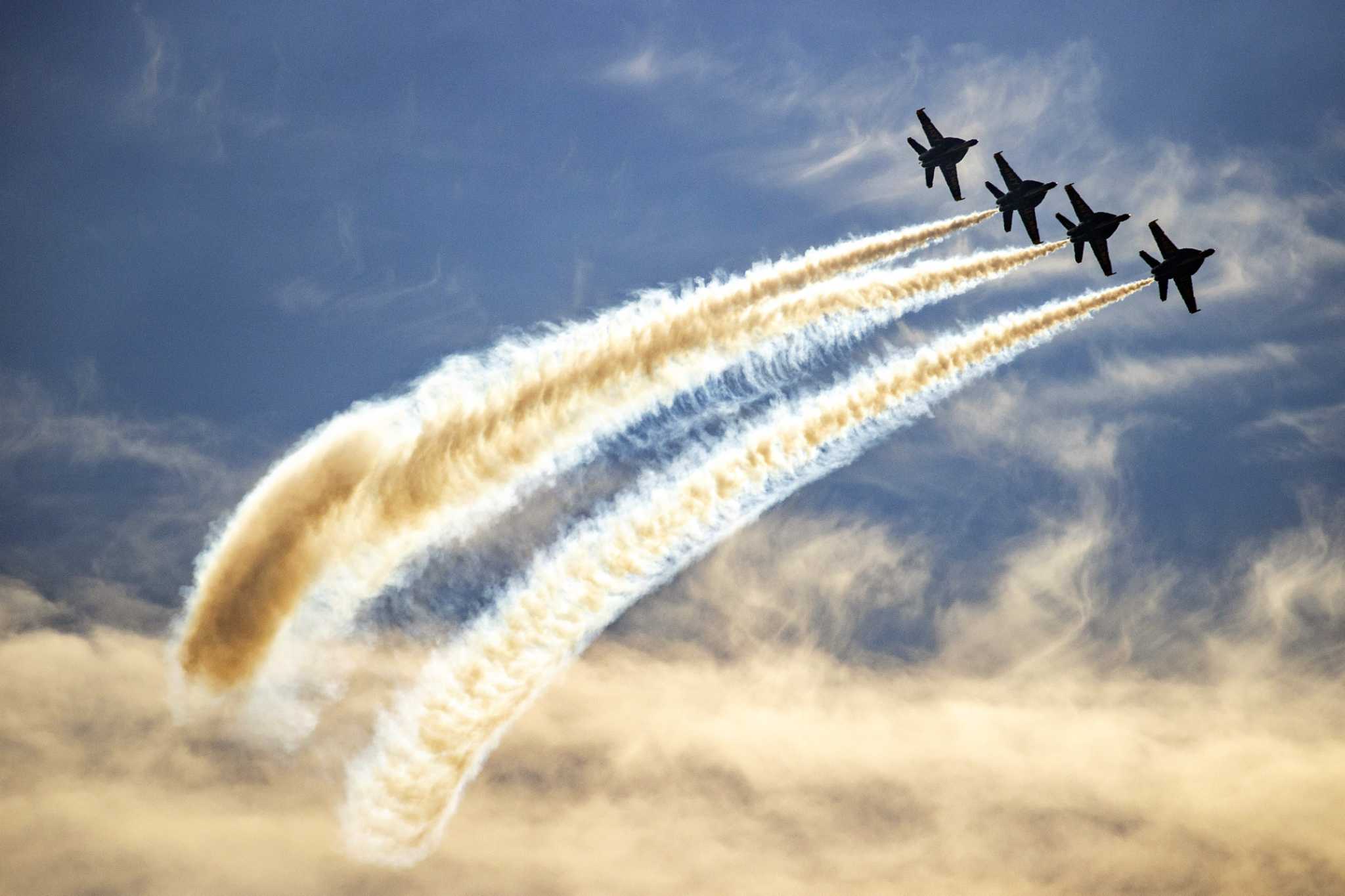A vibrant color landscape photograph captures an aerial demonstration by four fighter jets, reminiscent of the Blue Angels, performing in a clear mid-blue sky with light beige and white cloud accents. The top two-thirds of the image features this sky, while the bottom third displays a prominent beige-white cloud. Positioned in the top right-hand corner, the four jets fly in a staggered and diagonal formation, all facing the right. Three of the jets leave behind broadening trails of gold-tinted vapor with white highlights, blown slightly to the left by the wind, whereas the leading jet, located closest to the center, lacks such a trail. The jets are silhouetted black against the sky, creating a striking visual contrast, with the photorealistic style emphasizing the scene's dynamic realism.